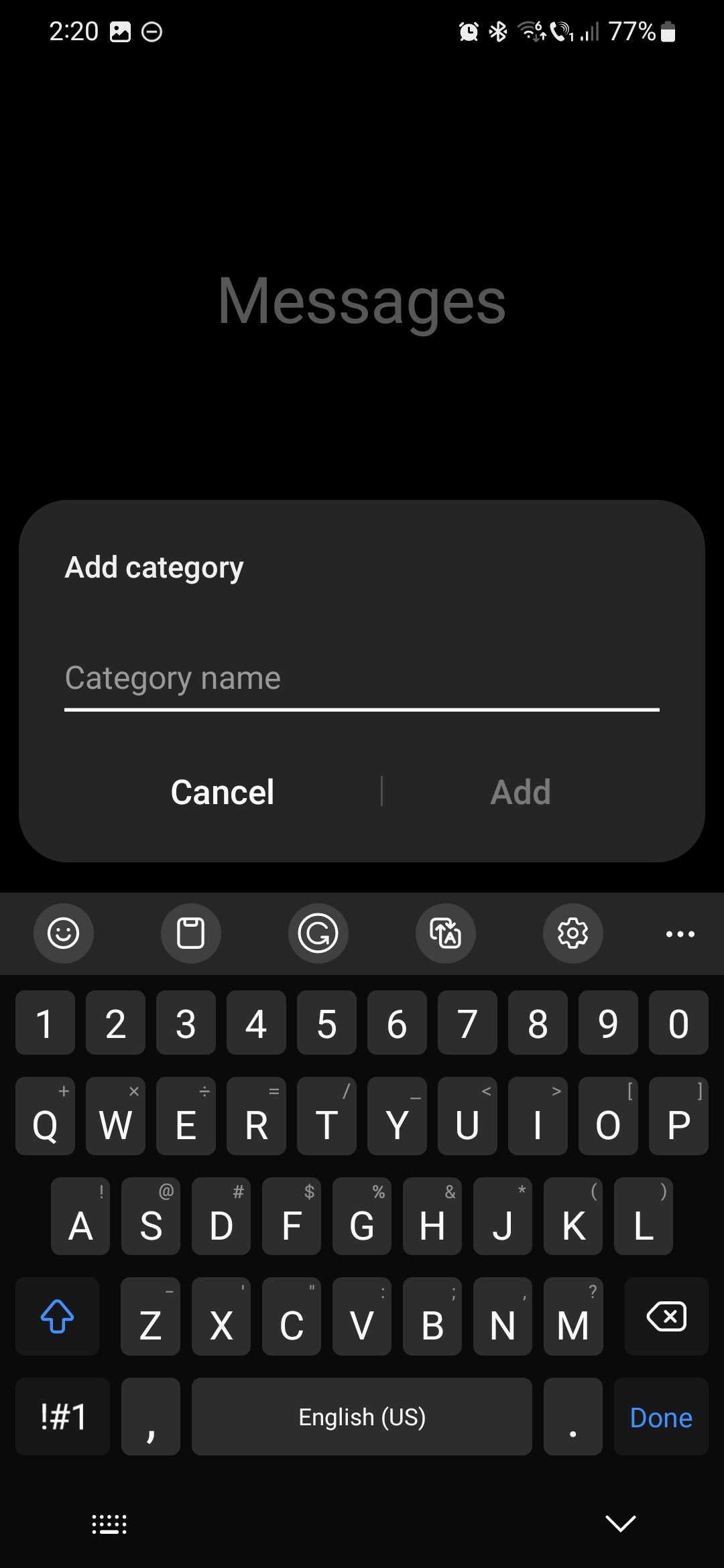Here’s a cleaned-up and detailed descriptive caption for the image:

---

The image appears to be a screenshot taken from a cell phone, showcasing an interface. In the upper left-hand corner, the number "220" is displayed. Below this, there is an image of a landscape. To the right, there is a circle with some dots inside it. Further to the right, several icons are present, including an alarm clock, Bluetooth symbol, a cell phone icon with two bars of signal, "77%", and a battery icon indicating the charge level is 77%.

The background of the image is black with white text. Lower on the screen, a grayed-out area prominently features the word "Messages" in large text. Beneath this, back in white text, the phrase "Add category" appears. Below this, in a lighter shade of grayish-white, is the text "Category name" followed by a thin horizontal white line. The words "Cancel" and "Add" are displayed with a slight vertical line separating them.

Further down, a virtual keyboard is visible. At the top of the keyboard are several symbols: a smiley face, a square icon, a refresh icon, the letter "A", a settings gear, and three vertical dots. The keyboard's top row shows numbers from 1 to 0. The next row includes the letters Q, W, E, R, T, Y, U, I, O, and P, each with additional symbols like plus, division, slash, underline, less than, greater than, right bracket, and left bracket above them. The following row consists of A, S, D, F, G, H, J, K, L, also featuring symbols such as exclamation mark, at sign, hashtag, dollar sign, percent, star, left parenthesis, and right parenthesis.

The third row of the keyboard has a shift/up arrow key, the letters Z, X, C, V, B, N, M, and a delete/backspace key marked with a left arrow and an "X." Above these letters, additional symbols include dash, apostrophe, quotation marks, colon, semicolon, comma, and question mark. On the bottom row, there is a key to switch to the symbols keyboard, labeled as "!?123", followed by a comma button, "English (US)" language button, period button, and the word "Done" in blue. There is also a small keyboard icon with a down arrow to the right.